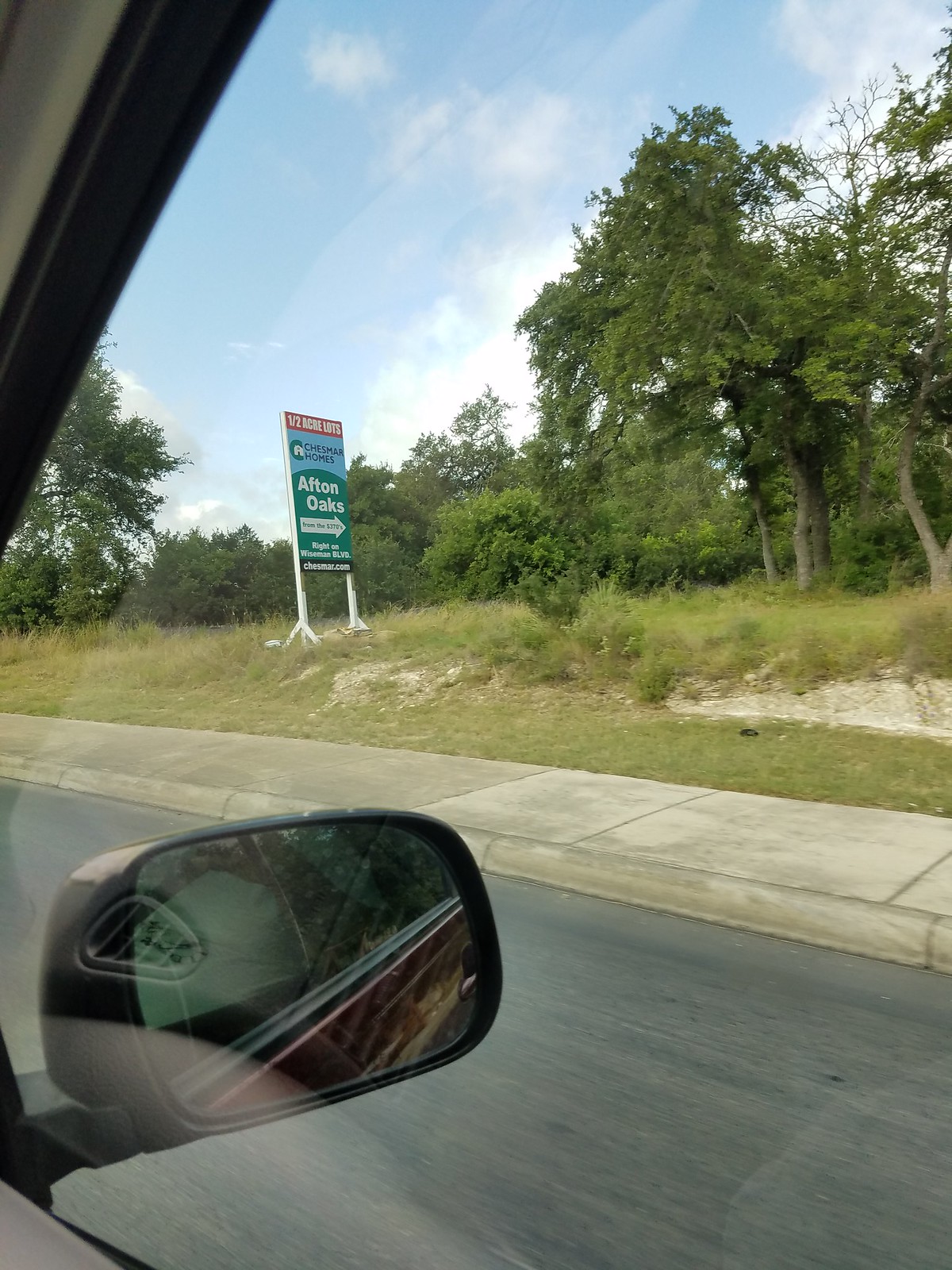This photograph, taken from the passenger side window of a car with a gray and black interior, captures a vivid roadside scene. The side mirror, reflecting part of the light gray seat and maroon red exterior of the car, frames a landscape bathed in sunlight under a blue sky dotted with white clouds. The road, dark asphalt streaked with light and dark gray, runs parallel to a light gray sidewalk that darkens in shaded and possibly wet areas. In the grassy expanse beyond the sidewalk, a sign with intricate details catches the eye. The sign reads "Afton Oaks," directing to the right with a white arrow on a green background. Additional text on the sign includes "Chesmore Mare Homes" and "Chesmore Mare.com" accompanied by decorative elements such as an ohm symbol inside a green circle, all presented on various colored backgrounds including brown, red, and black. Surrounding the area are alternating patches of light and dark green grass, a dug-up section with gray rocks, and lines of trees and hedgerows blending shades of green. The photograph encapsulates a serene, wooded scene adjacent to urban infrastructure, juxtaposed with the reflective surfaces of the car's interior.